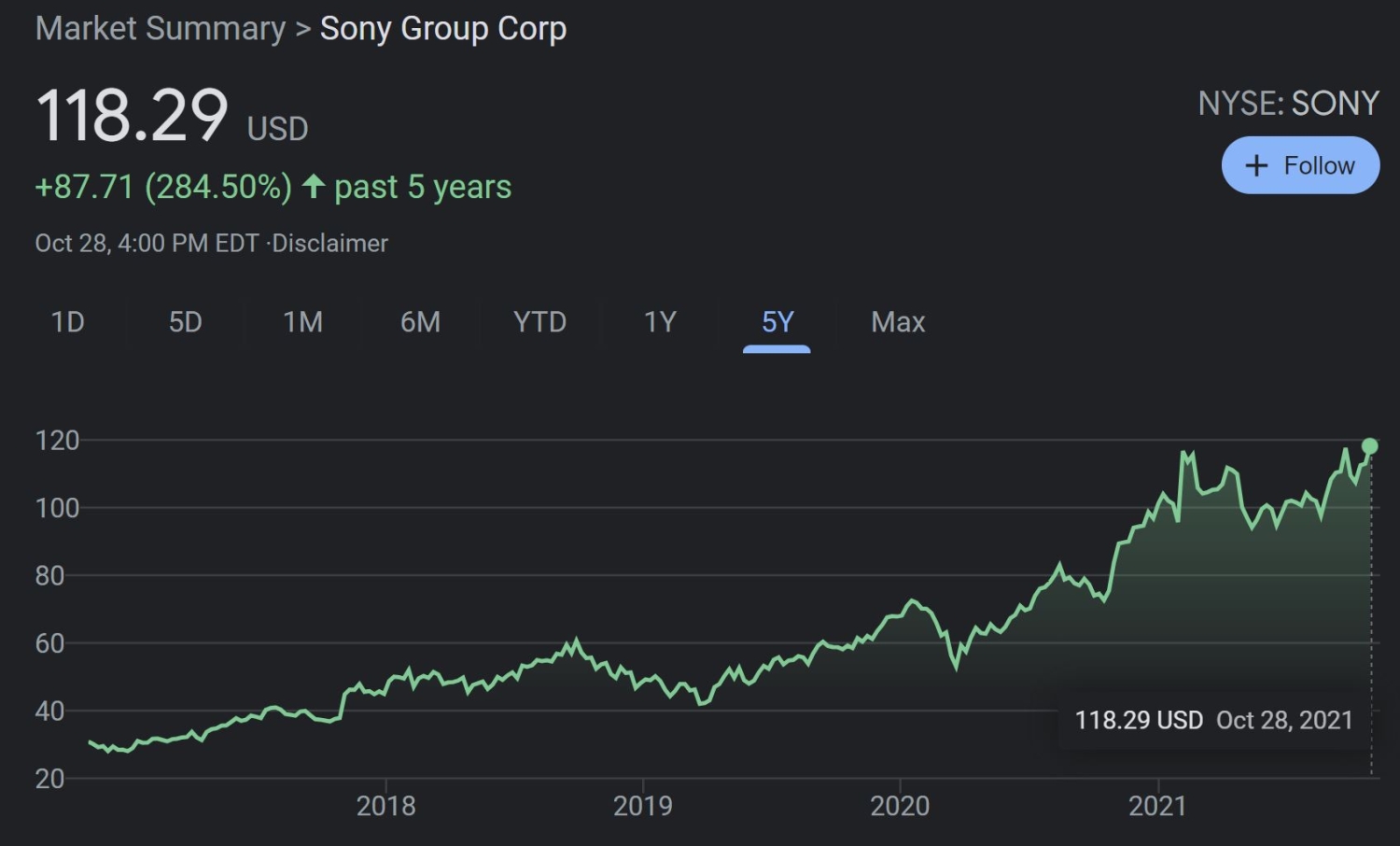This image provides a detailed market summary for Sony Group Corp. Positioned at the upper left corner, the title "Market Summary" is followed by a "greater than" symbol pointing to "Sony Group Corp." The stock price is listed at $118.29 USD. Below that, a notable increase of $87.71 (or 284.50%) is indicated, with an up arrow signifying growth over the past 5 years. Further details note the timestamp as "October 28th, 4 PM EDT," accompanied by a small dot and the word "disclaimer."

The central part of the image features a chart offering various time frame options such as 1 day, 5 days, 1 month, 6 months, year-to-date, 1 year, 5 years, and max. The 5-year time frame is selected, highlighting a consistent upward trend in Sony's stock price from 2018 to 2021.